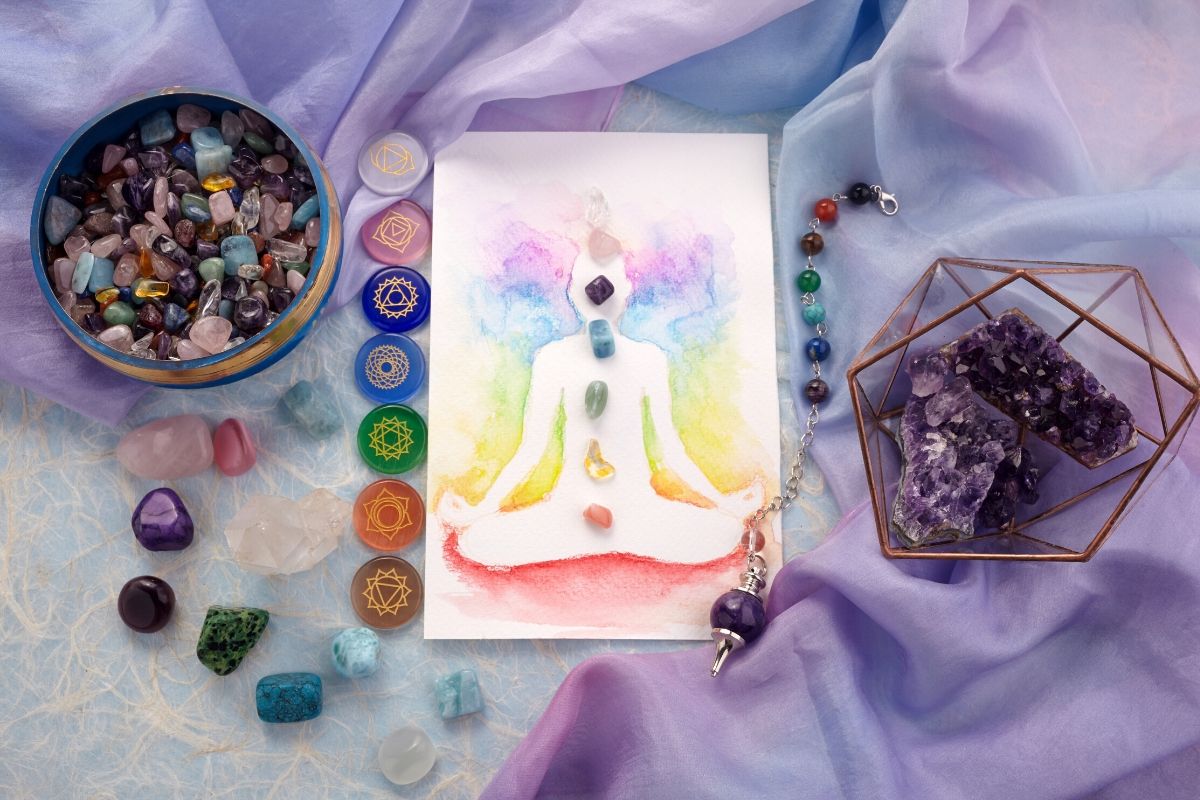The image showcases a serene and spiritually-themed arrangement centered on a watercolor painting of a person meditating, seated in a cross-legged lotus position with hands raised in a typical meditative pose. The figure itself is uncolored but radiates an aura comprised of rainbow hues. Six small, multicolored gemstones, reminiscent of chakra colors, are placed along the center line of the figure, contributing to the sense of tranquility and spiritual alignment.

Adjacent to the painting on the right side is a large, dark purple crystal resembling a geode, next to a bracelet adorned with colorful healing beads. Further to the right is an angular bowl filled with purple stones. To the left of the painting are various stones with intricate engravings and a vibrant blue bowl filled with a multitude of small, colorful gems and stones.

The entire arrangement is set atop a luxurious, silky fabric that transitions from light purple to dark blue, serving as a plush and calming backdrop to the assortment of healing crystals, stones, and beads spread across the scene.